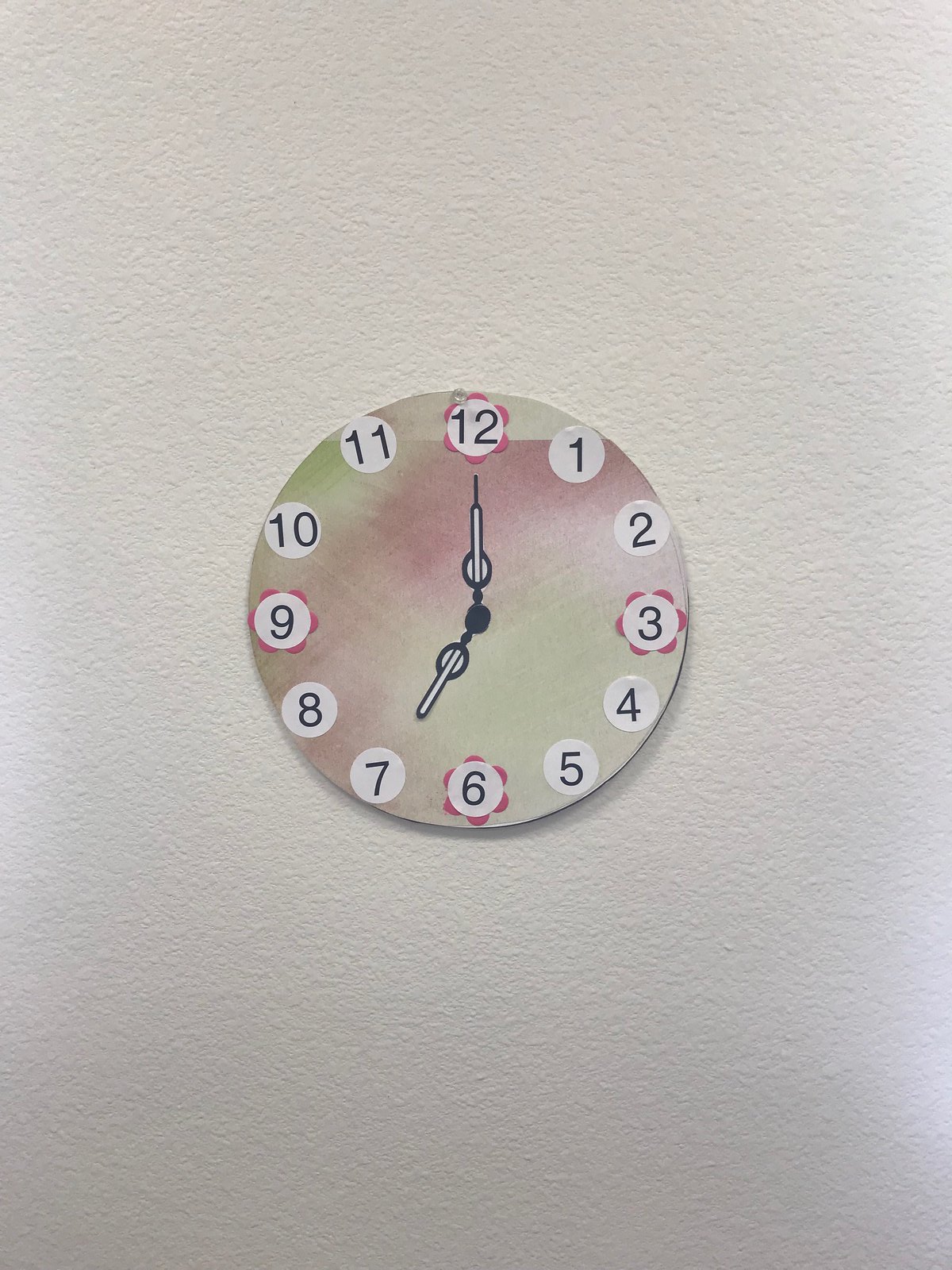This photograph features a handcrafted clock mounted on a textured white stucco wall. The clock, appearing as an arts and crafts project possibly made out of cardboard, boasts a background with watercolor-like brush strokes in lime green and light reddish colors. Each number from 1 to 12 is depicted in black font on white circular discs. Notably, the numbers 12, 3, 6, and 9 are adorned with scalloped edges resembling pink or red flower petals. The clock hands, designed to appear three-dimensional and decorative, are color-coordinated in black and white, and indicate the time as 7 o'clock. The clock is hung up by a clear pushpin located right above the 12, and there is no second hand present. The remaining portion of the white stucco wall is left blank.